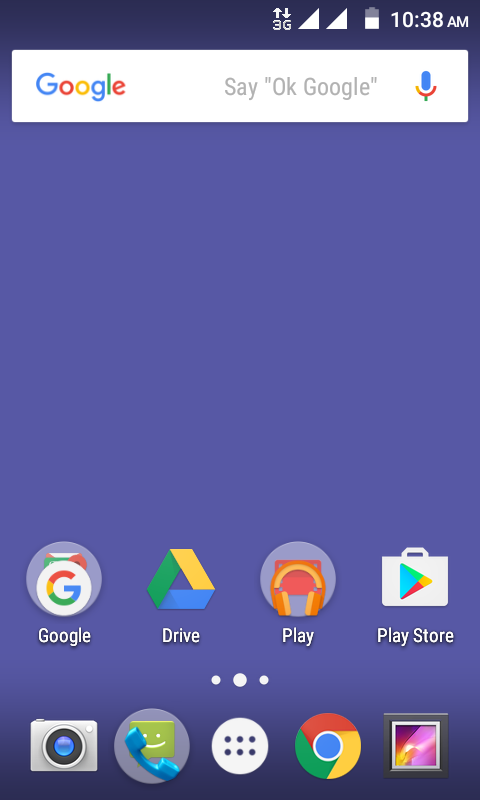The image showcases a tall rectangular layout with a predominantly purple background. At the top, spanning almost the entire width from left to right, is a wide white rectangle containing the Google logo, which consists of a capital blue 'G', a small red 'o', a yellow 'o', a blue 'g', a green 'l', and a red 'e'. On the far right end of this white bar, there is a microphone icon. In the center of this bar, written in gray letters, are the words "Say, 'OK Google'", with "OK Google" enclosed in quotation marks.

Below the white bar lies a large blank space filled with the purple background. At the bottom of the image, there are two rows of icons. The top row contains four icons, each labeled in white text. From left to right, they are:
1. "Google" with a circular logo featuring a capital 'G' in red, yellow, green, and blue.
2. "Drive" with a triangular logo resembling folded ribbon, colored yellow on the right, green on the left, and blue at the bottom.
3. "Play" with a gray circle featuring a design in orange and red that somewhat resembles a table.
4. "Play Store" with an icon of a white suitcase containing overlapping triangles in blue, red, and yellow, with the blue triangle on top.

The bottom row includes five more icons:
1. A camera icon with a gray body and a black circle center with a blue circle inside it.
2. A gray circle featuring a lime green square with a white smiley face, plus a blue telephone receiver angled at 45 degrees in front of the square.
3. A white circle with two rows of three purple dots each.
4. Another Google logo, this time with a blue circle at the center surrounded by an outer circle that is red at the top, yellow on the right, and green on the left.
5. An icon resembling a computer monitor or TV screen, outlined in light gray with the interior square displaying pink, yellow, and dark purple colors.

Each detail in the image has been meticulously described, providing a vivid understanding of its composition and the elements within it.